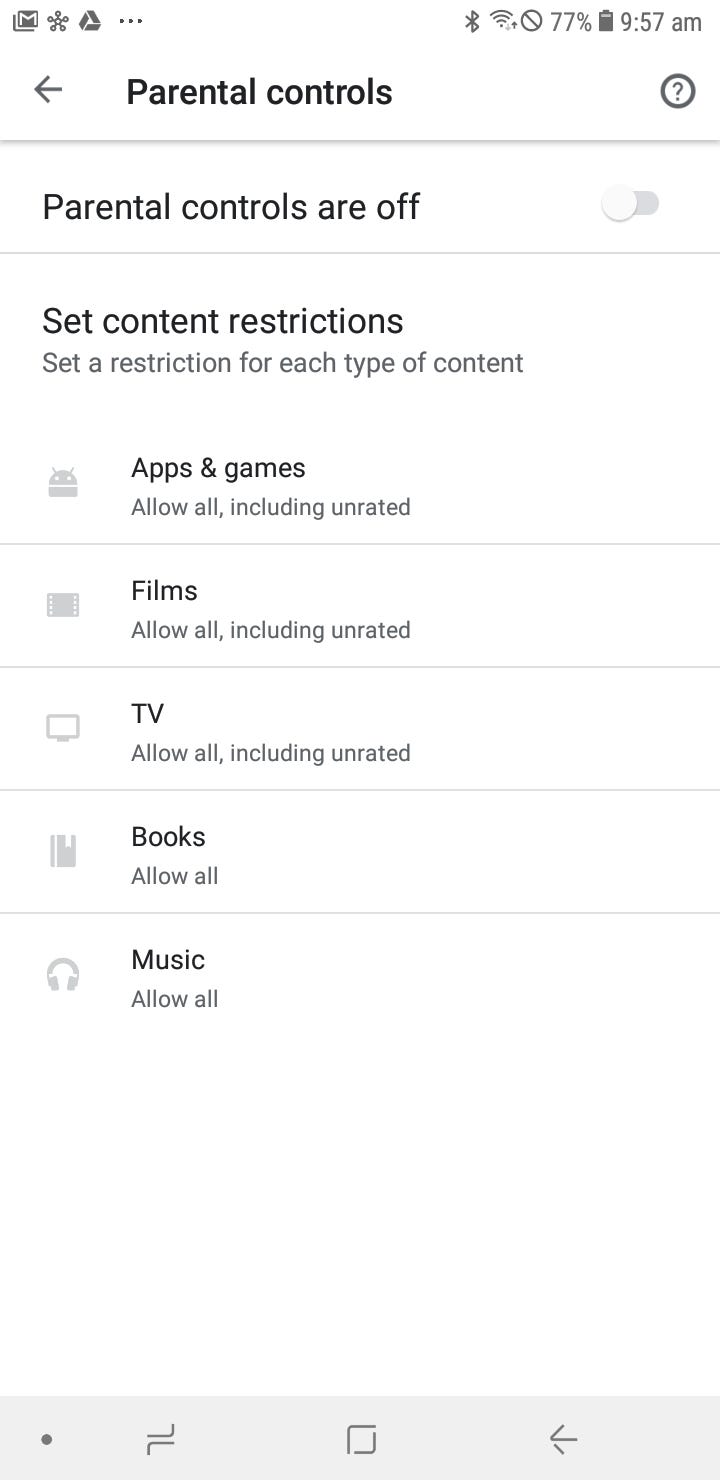The image depicts the settings menu for parental controls on an Android device. The top left corner displays a Gmail logo, indicating it's an Android interface. To the right of the Gmail logo, there is an icon resembling a star or flower, followed by the Google Drive logo. Adjacent to these icons are three vertical dots, commonly known as the "more" menu.

Prominently displayed in bold black lettering is the title "Parental Controls" with a left-pointing arrow beside it, indicating a back navigation option. Opposite the arrow, on the top right, is a question mark encircled in a bold gray outline, signifying a help or information section.

A light gray shadowed divider separates the header from the main content, under which it states "Parental controls are off" with a switch available to toggle the controls on. Below this, a thin light gray divider introduces the section labeled "Set content restrictions" in black lettering. Underneath, smaller light gray text explains, "Set a restriction for each type of content."

Listed are various content categories:
- Apps and games, indicated with the Android icon, are set to "Allow all, including unrated."
- Films, represented by a film icon, set to "Allow all, including unrated."
- TV shows, symbolized by a monitor icon, also set to "Allow all, including unrated."
- Books, shown with an icon that includes a bookmark, set to "Allow all."
- Music, represented by headphones, set to "Allow all."

At the bottom of the menu is a light gray strip featuring a bullet point on the far left side, followed by an icon that resembles a wrench or an upward-downward line, a square icon, and an arrow pointing to the left, which likely functions as additional navigation or settings options.